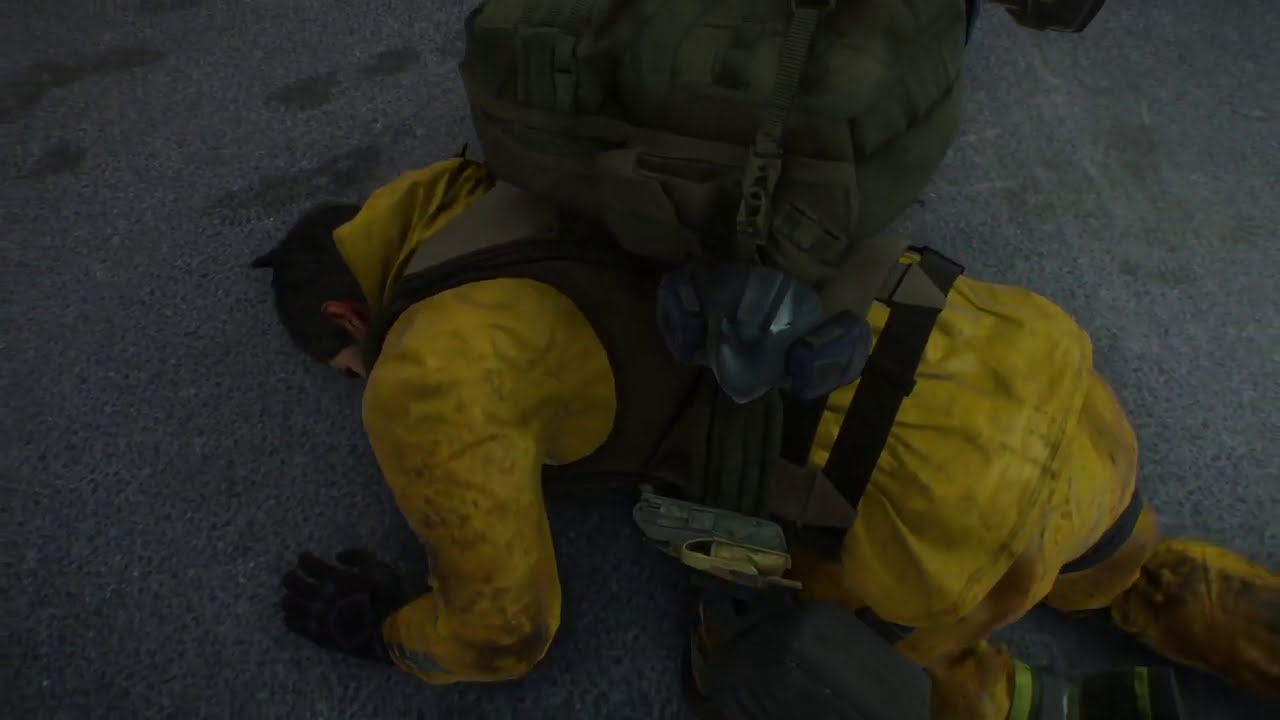The image depicts a man wearing a bright yellow uniform that resembles a fireman's gear, complete with a yellow long-sleeved coat and yellow pants. He is lying face down on a weathered gray pavement, which has small oil spots above his head. The man is equipped with black mechanics gloves, safety shoes, and a black belt with a vest. A large, heavy green military-style backpack is strapped to his back, with an additional support brace to help carry the weight. His left arm is extended outward and bent at the elbow, with the left side of his face, including his ear, slightly visible as he rests his head on the ground. The scene appears realistic but could also be mistaken for a screenshot from a video game due to its detailed, dramatic composition.